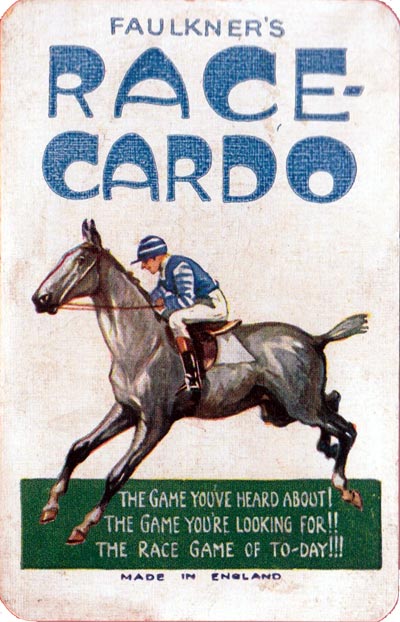The image appears to be a vintage cover, possibly dating from the early to mid-20th century, for the box of a game titled "Faulkner's Race-Cardo." At the very top, centered in modernist sans serif blue lettering, is the name "Faulkner's." Directly beneath it, in significantly larger, decorative, and bubbly lettering with thick, rounded tops, are the words "Race" and "Cardo." The primary illustration features a jockey riding a gray-black horse, both oriented almost entirely to the left. The jockey is dressed in a blue-striped hat, a blue shirt with horizontal stripes on the sleeves, white tight pants that reach just below the knees, and black boots. A field of green stretches across the bottom of the image, with white text displaying three lines of enthusiastic promotional phrases: "The game you've heard about!" (one exclamation point), "The game you're looking for!!" (two exclamation points), and "The race game of today!!!" (three exclamation points). Below the green strip, in black capital letters, is the phrase "MADE IN ENGLAND." The weathered paper and rounded corners of the image add to its vintage appeal.